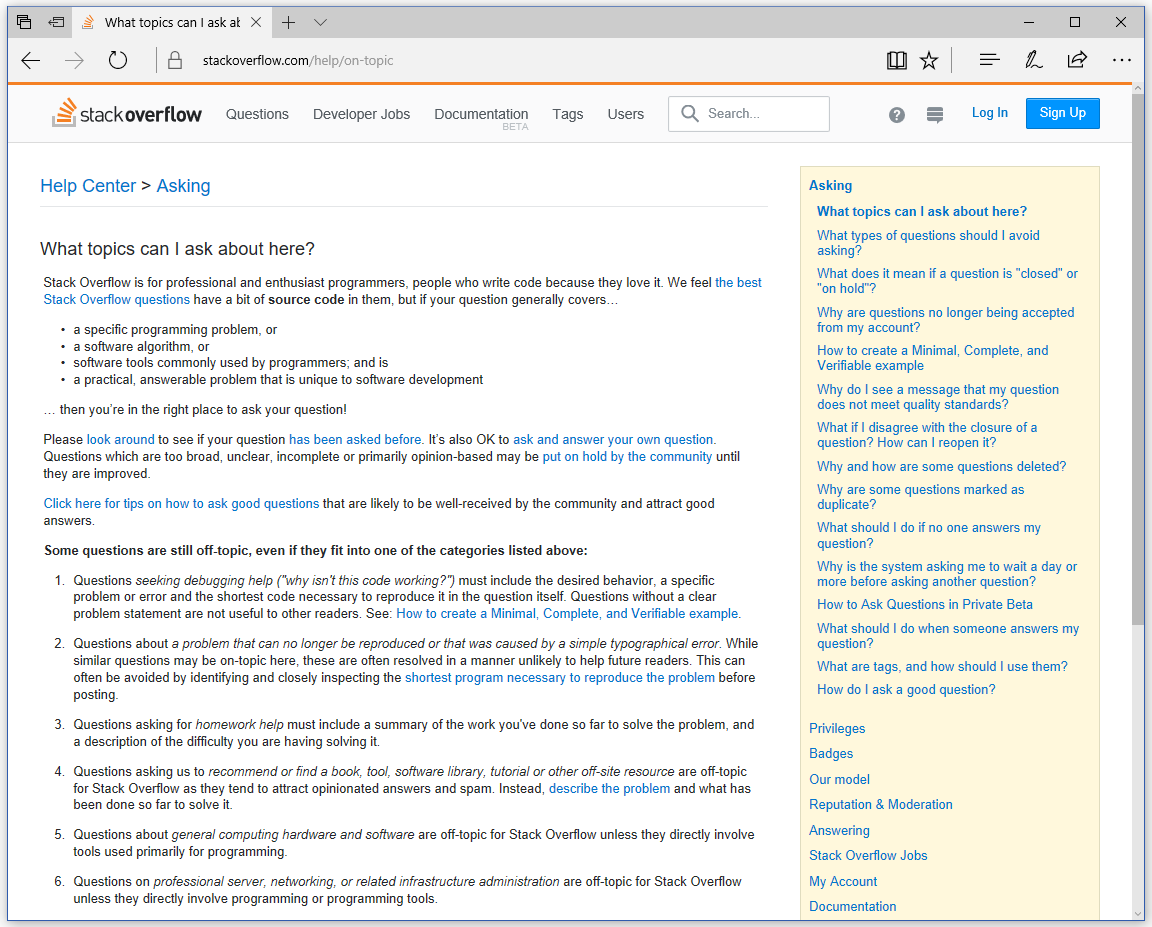The image appears to be a screenshot of someone's computer screen displaying the Stack Overflow website. 

At the top of the screen, there is a gray browser interface with a tab titled "What topics can I ask at...". Below this, you see navigation controls including a back arrow, a refresh button, and the website URL, stackoverflow.com.

The main content of the image is divided into two sections: 
- The left section, predominantly white, begins with the Stack Overflow logo. Below the logo, there are navigational links labeled "Questions," "Developer Jobs," "Documentation," "Tags," "Users," and a search bar. Located further to the right are "Sign Up" and "Log In" buttons.
- Directly under these is a "Help Center" header with the subheading "What topics can I ask about here?". This section includes detailed guidelines on acceptable question topics, displayed in a paragraph followed by bullet points. The bullet points list:
  1. A specific programming problem
  2. A software algorithm
  3. Software tools commonly used by programmers
  4. A practical, answerable problem unique to software development

Beneath the listed points, a warning states, "Some questions are still off-topic even if they fit into one of the categories listed above," followed by a list of six specific points.

On the right side of the image, there is a yellow column labeled "Asking." This column presents several questions followed by sections titled "Privileges," "Badges," "Our model," "Reputation," and "Moderation." Lower down, it includes links to "Answering," "Stack Overflow," "Jobs," "My Account," and "Documentation."